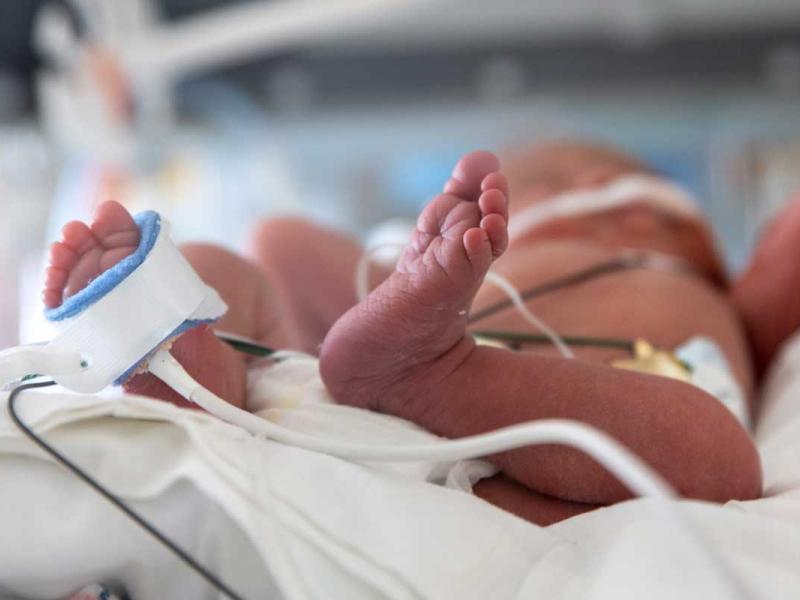The image captures a newborn baby in a hospital setting, likely in an ICU. The large, almost square-shaped photograph is horizontally aligned, with a blurred background indicating the indoor hospital environment. The focus of the image is on the baby's tiny, delicate feet, which are sharply detailed, showing all the little wrinkles. The right foot, located on the left side of the image, is wrapped in a monitor cuff with blue padding and a white exterior, from which a white cord extends at a downward angle towards the lower right of the picture. The infant, lying on a wrinkled white sheet atop a clear hospital bed, is dressed in a diaper but no other clothing, and is connected to various medical tubes and wires. A white tube is visible near the baby's mouth and nose, likely for breathing assistance, while black wires can be seen across its stomach. This poignant image highlights the vulnerability and preciousness of new life, being carefully monitored and cared for in a medical setting.